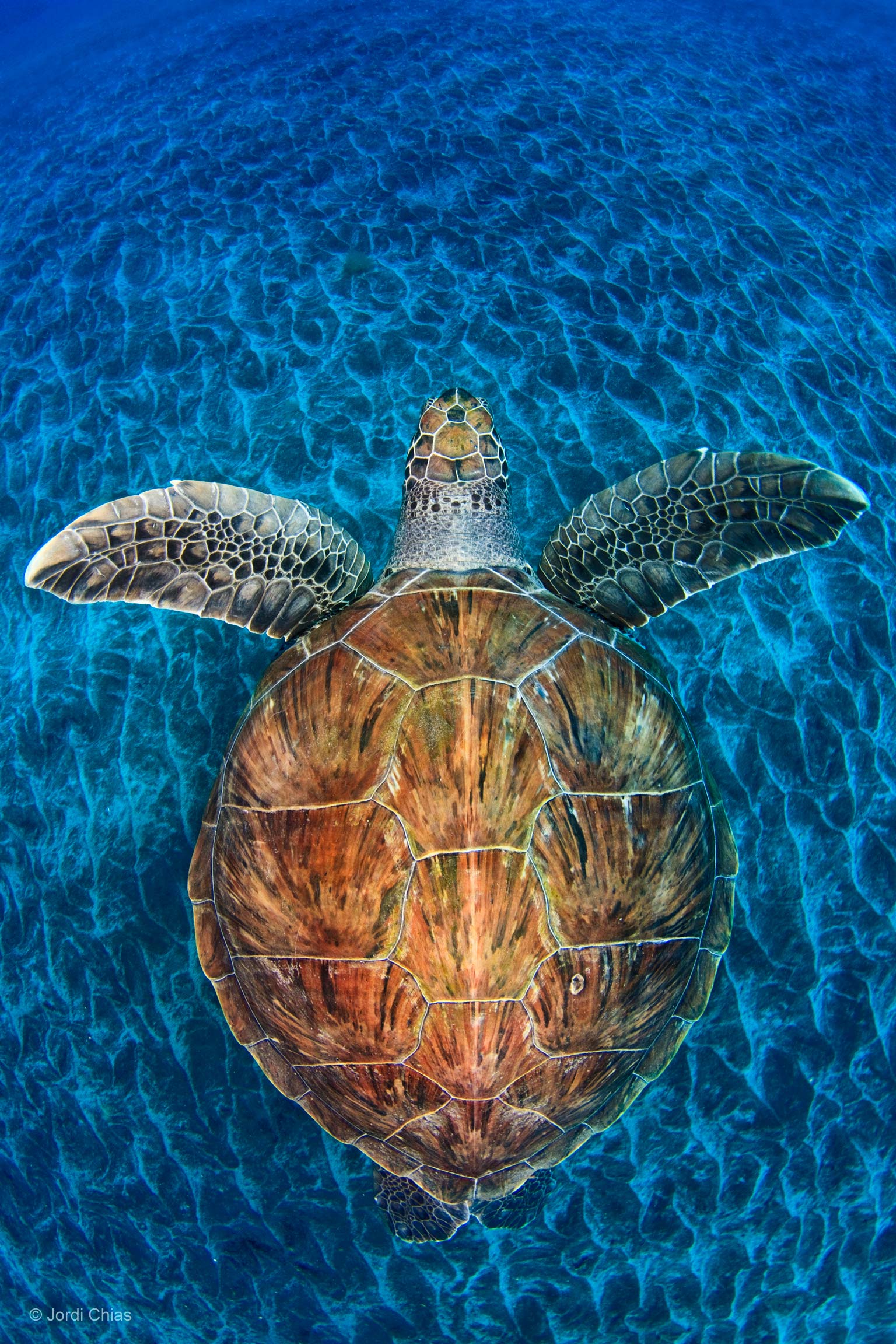This detailed image depicts a majestic sea turtle swimming gracefully in a vibrant cerulean blue ocean. Dominating the center of the image, the turtle's large, symmetrical brown shell, accented with darker stripes, stands out against the deep blue background. With its two front fins outstretched to each side, the turtle appears to be gliding effortlessly through the water. The scene gives the impression of looking up from the ocean floor, observing the turtle from below as its head faces away from the viewer towards the top of the image. The texture of the turtle's fins is distinctly gray and alligatored, adding to the lifelike quality of the portrayal. Small wave-like patterns can be seen in the water, enhancing the dynamic feel of the scene. In the bottom left corner, there is a watermark that reads "Jordy Chias," suggesting the artist or photographer behind this captivating work.